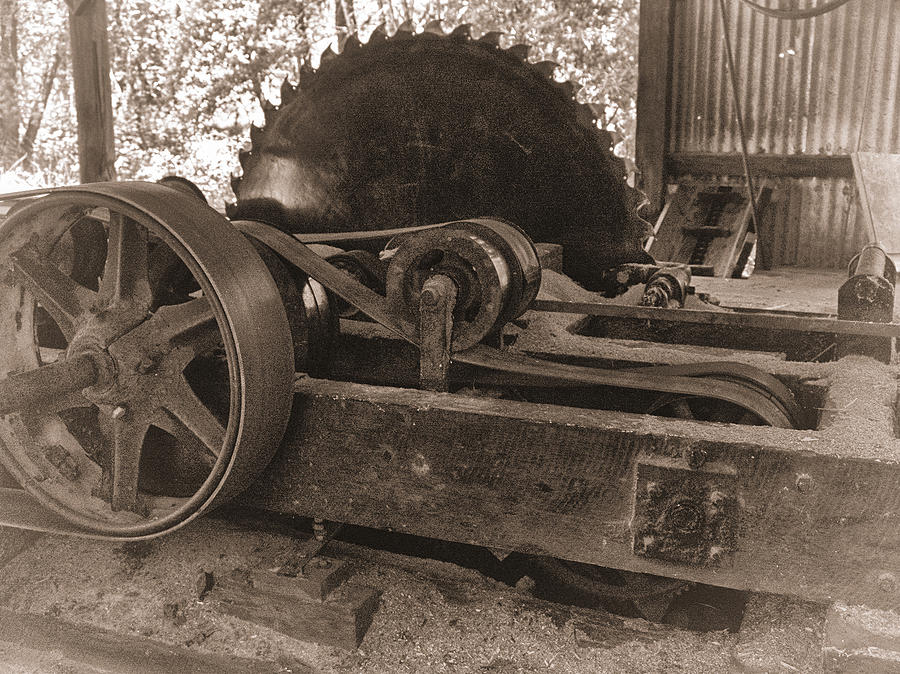This rectangular, black and white photograph, which has a patina-like brownish tint, captures an old-time sawmill scene. The sawmill, an intricate metal and wooden machinery, dominates the image. Central to the composition is a monumental, black saw blade with sharp, pointy teeth. In the foreground, there is a system of belts and pulleys: a wheel on the front left connects via belts to other wheels in the middle of the machine. The sawmill sits upon sturdy wooden beams resting on a gravel-strewn ground. Sawdust is scattered across both the blade and the floor, evidence of its use. The background reveals trees on the left, suggesting an open-air or partially enclosed shed, which is reinforced by a corrugated metal wall visible on the right. The entire setup exudes a sense of rustic functionality, reflective of an era gone by.